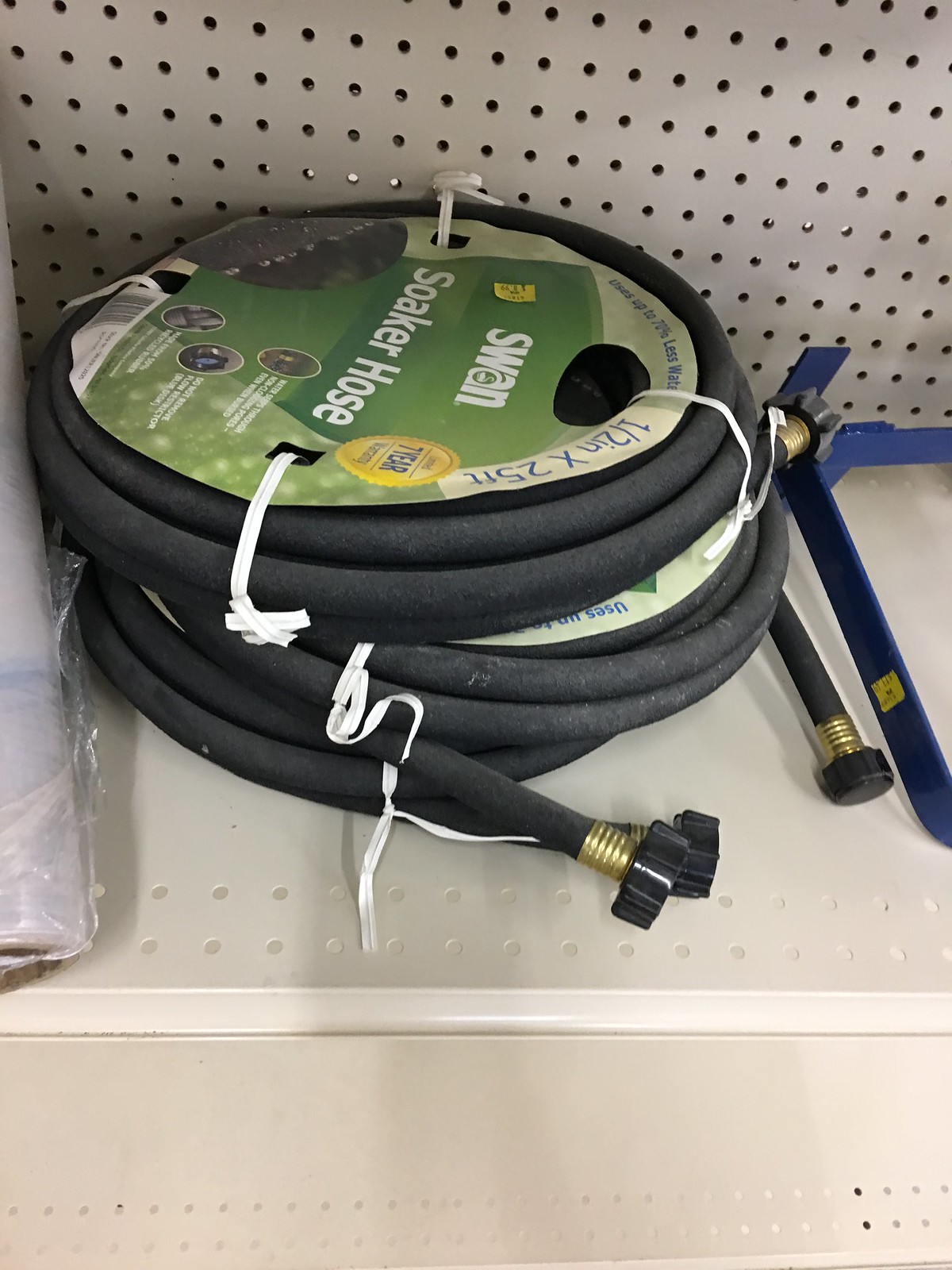This photograph captures a display of coiled black fabric garden hoses, branded as "Swan Soaker Hose", arranged on a perforated beige metal shelf in what appears to be a hardware store. The shelf features numerous small holes for adjustable shelving. The hoses are neatly stacked, though they appear slightly worn, and are fastened with green, white, and blue labels indicating their dimensions: half-inch in diameter and 25 feet in length. These labels also provide usage instructions. Visible on the shelf are two hoses, with their connectors peeking out. To the right, a blue metal object is partly visible, while to the left, a plastic-wrapped item, resembling shrink wrap, can be seen.